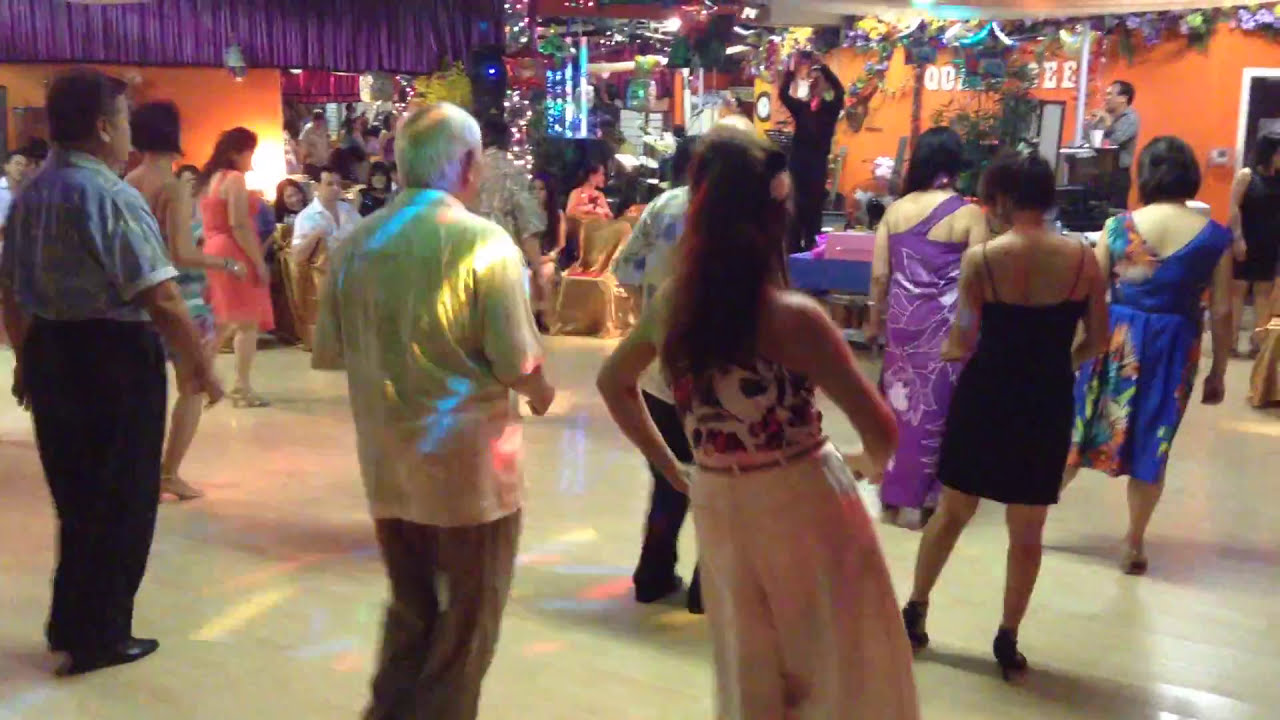The image features a lively group of fewer than 100 elderly individuals, both men and women, engaged in a line dance on a wooden dance floor, their backs turned to the camera. The scene appears to be in a vibrant, indoor setting, possibly an auditorium or a common area of a recreation center, decorated festively with banners, celebratory pictures, and a purple pleated valance visible in the top left corner. The participants, dressed in an array of colorful dresses, shirts, and pants, are spread out with space between each person, suggesting a synchronized dance similar to the Macarena. Dance floor lighting highlights the dancers' bodies, adding to the festive atmosphere. Towards the top center of the image, a person dressed in all black is seen with hands raised, seemingly capturing a photograph of the group. In the backdrop, partly obscured, are letters and celebratory decorations, including a star balloon, hinting at a celebratory event. The environment and the crowd's joyful engagement suggest the setting could be a party, wedding, or celebration within a retirement or senior citizen’s home.